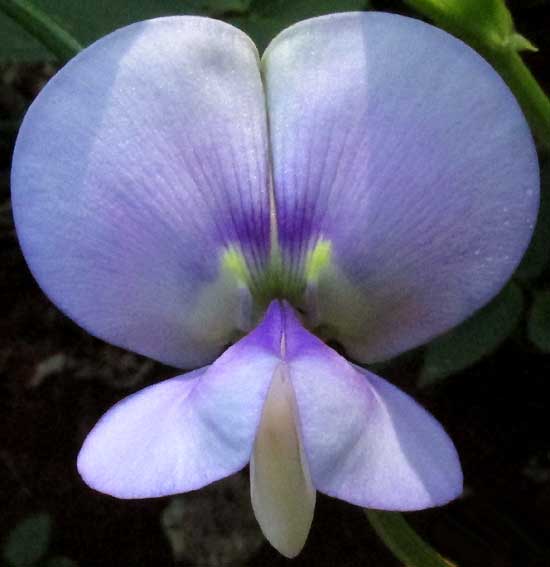This detailed close-up image appears to be a macro shot of a stunning purple orchid. The flower's unique structure creates an almost lifelike appearance, resembling a face or an insect. The top part of the image features two large, rounded petals with edges that fade to a nearly white color. As these petals extend toward the center, their color deepens into a rich and dark purple. At the middle of the flower, there's a bright yellow patch that looks strikingly like big eyes. Below this, additional petals spread out in such a way that they resemble a mouth or insect mandibles. Sprinkles of yellow further enhance the lifelike quality of the flower. The background is dark, characterized by shades of black and green, with visible stems and leaves that place the flower in a natural outdoor setting, possibly in front of a tree. Overall, the flower's orientation appears straightforward, directly facing the camera, capturing its intriguing and almost surreal beauty.